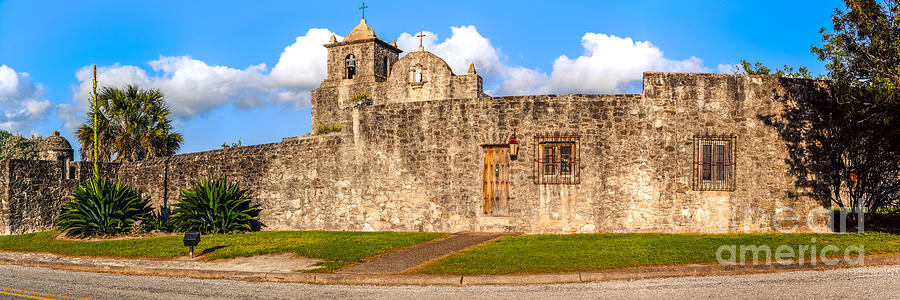The photograph features a historic mission or abbey with a castle-like appearance, characterized by a wide, tall wall made of interlocking bricks and stones in shades of black, brown, and light brown. Central to the image, the wall includes two barred windows and a small, sturdy wooden door accentuated by a lamp to its right. A gray gravel walkway, bordered by a lush green lawn, leads up to the door from a gray asphalt road marked by a double yellow line, highlighting its lanes.

Behind the main wall, two interconnected buildings rise, each distinguished by unique roof structures. The left building has a block shape with a triangular roof crowned by a cross, while the right building features an arch-shaped top also adorned with a cross. An additional tower equipped with a lower-case T-shaped cross stands prominently against a backdrop of vibrant, blue sky filled with fluffy white clouds.

The landscape in front of the wall includes a freshly cut grassland, two short bushes to the left, and a gravel path flanked by green lawns. There's a black spotlight set into the lawn intended to illuminate the tower at night. The upper right corner of the image features part of a tree, and an overlaid text that partially reads "America" hints at the photograph's historical or cultural context.